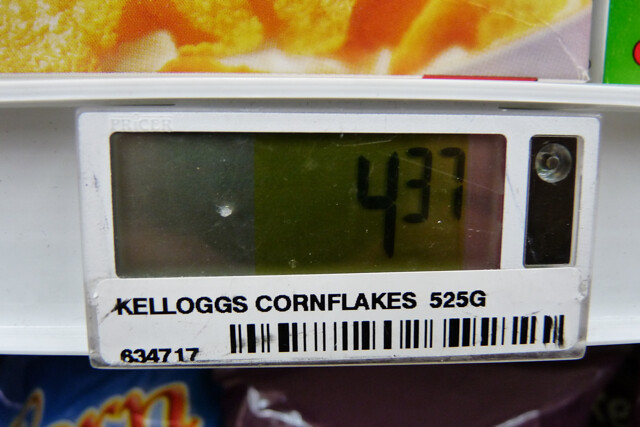The image is a detailed, landscape-style photograph taken inside a grocery store, centering on a digital price tag for a box of cereal. The main focal point is the LED screen displaying the price of $4.37, set against a green background. Below the screen, in black lettering, it reads "Kellogg's Corn Flakes, 525 grams," accompanied by a barcode and an item number "634717" situated at the bottom left of the barcode. The upper portion of the image reveals the slightly cut-off bottom of a Corn Flakes box, showing a few golden flakes. Toward the bottom of the image, portions of other cereal boxes are visible: a blue-colored box in the left corner and a purple-colored box in the middle to the right. The image captures the white structure of the shelf, emphasizing the digital nature of the price display, which is indicative of the modern grocery store setting.